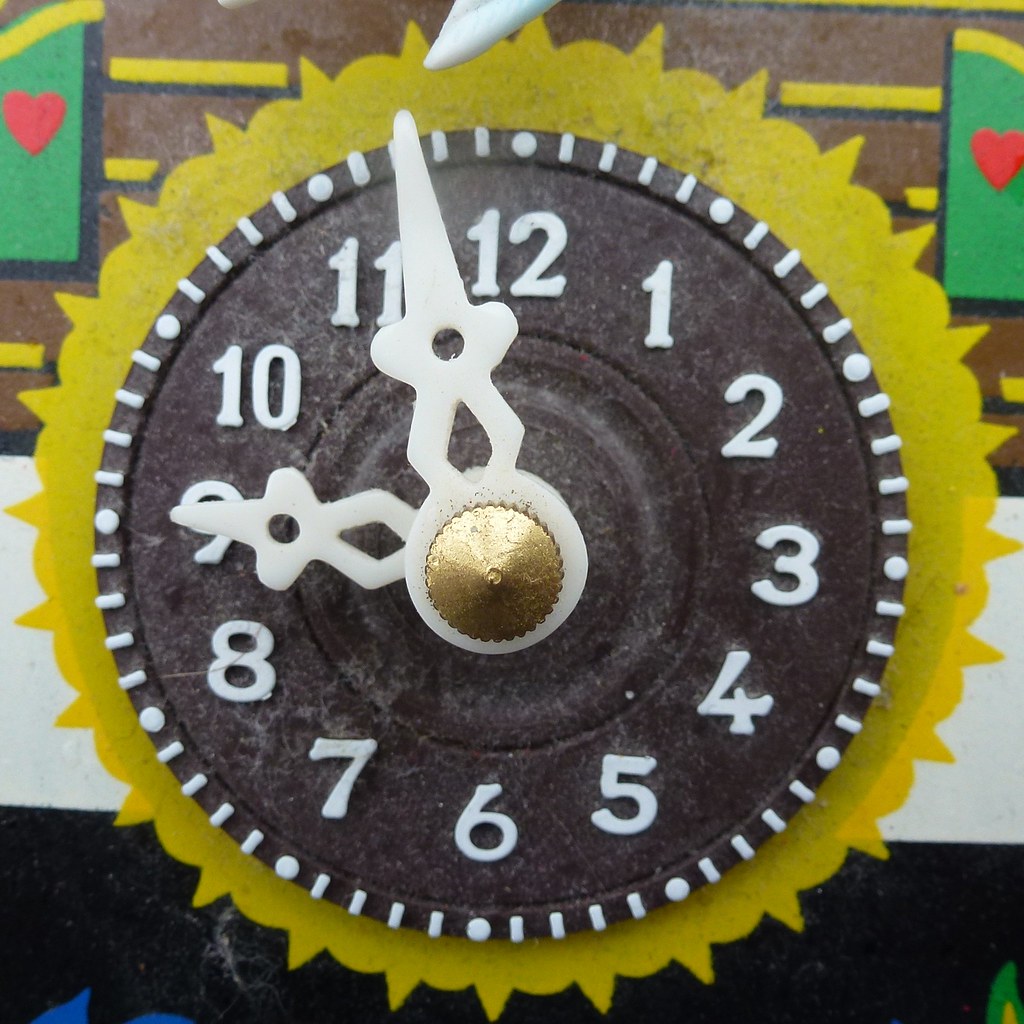This image features a round clock positioned prominently in the foreground. The clock has a brownish hue, complemented by white numerals marking each hour. Along the edge of the clock face, white dots denote individual hours, with smaller white lines in between for minute increments. The hands of the clock indicate the time as 8:58. Surrounding the clock is a striking yellow design resembling the rays of the sun, giving the impression that the sun is radiating from behind it.

The background is a complex tapestry of colors and patterns, featuring shades of brown and intersecting yellow lines, providing a sense of depth and texture. Adding a touch of whimsy and charm, there are sections of green positioned in the upper left and right corners, each adorned with a small red heart at its center. These details create a rich and captivating visual narrative, though the precise setting of the clock—whether mounted on a wall or affixed to an object such as a toy train—remains delightfully ambiguous.